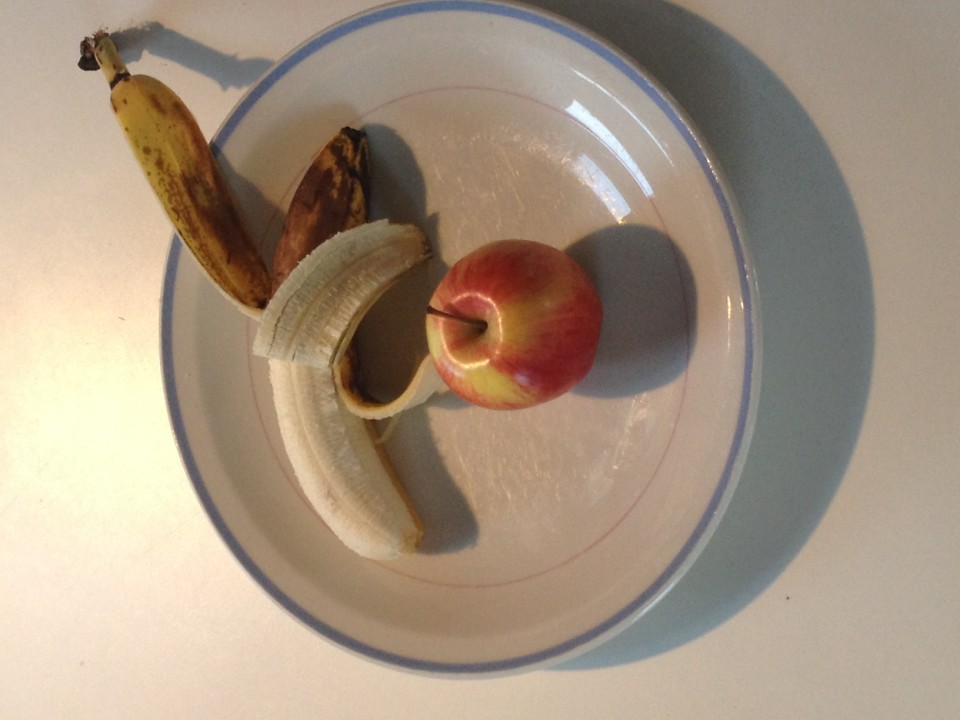The image features a worn, white dining plate adorned with a delicate blue edge and a thin, light brown or black inner circle. The center of the plate is dotted with numerous light cut marks, indicative of years of use. On the plate rests a light red apple with yellow tinges, complete with its stem. Beside the apple, on the left, is a partially peeled banana. The banana's peel is heavily marked by brown spots, though some yellow remains, and its stem is notably brown. The unpeeled portion of the banana’s tip is dark brown, while its interior appears near perfect, save for a slight bruise. The lighting, coming from the left side, casts a distinct three-bar reflection on the plate and generates a shadow to its right.